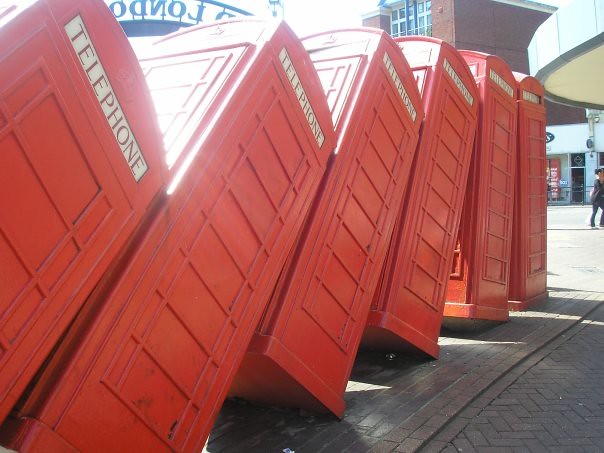The photograph captures a striking scene featuring six life-sized, solid plastic replicas of iconic British red telephone booths, known for their characteristic charm. These replicas are meticulously designed, complete with indented window contours devoid of glass and topped with white rectangular strips that bear the red-lettered word "TELEPHONE." The booths are arranged in a dramatic, domino-like formation, tilted and leaning into one another from left to right, culminating with the last booth standing upright at the far right edge of the frame.

The telephone booths are positioned on a brick platform, which transitions into a neighboring stone pathway designed with distinct zigzag patterns in gray bricks. This artistic display or exhibit is set against a backdrop of a brick building, contributing a historical texture to the scene. Walking figures on the cement pathways in the background add a layer of life and movement to the photograph, blending modern pedestrian activity with the timeless allure of the red telephone booths.